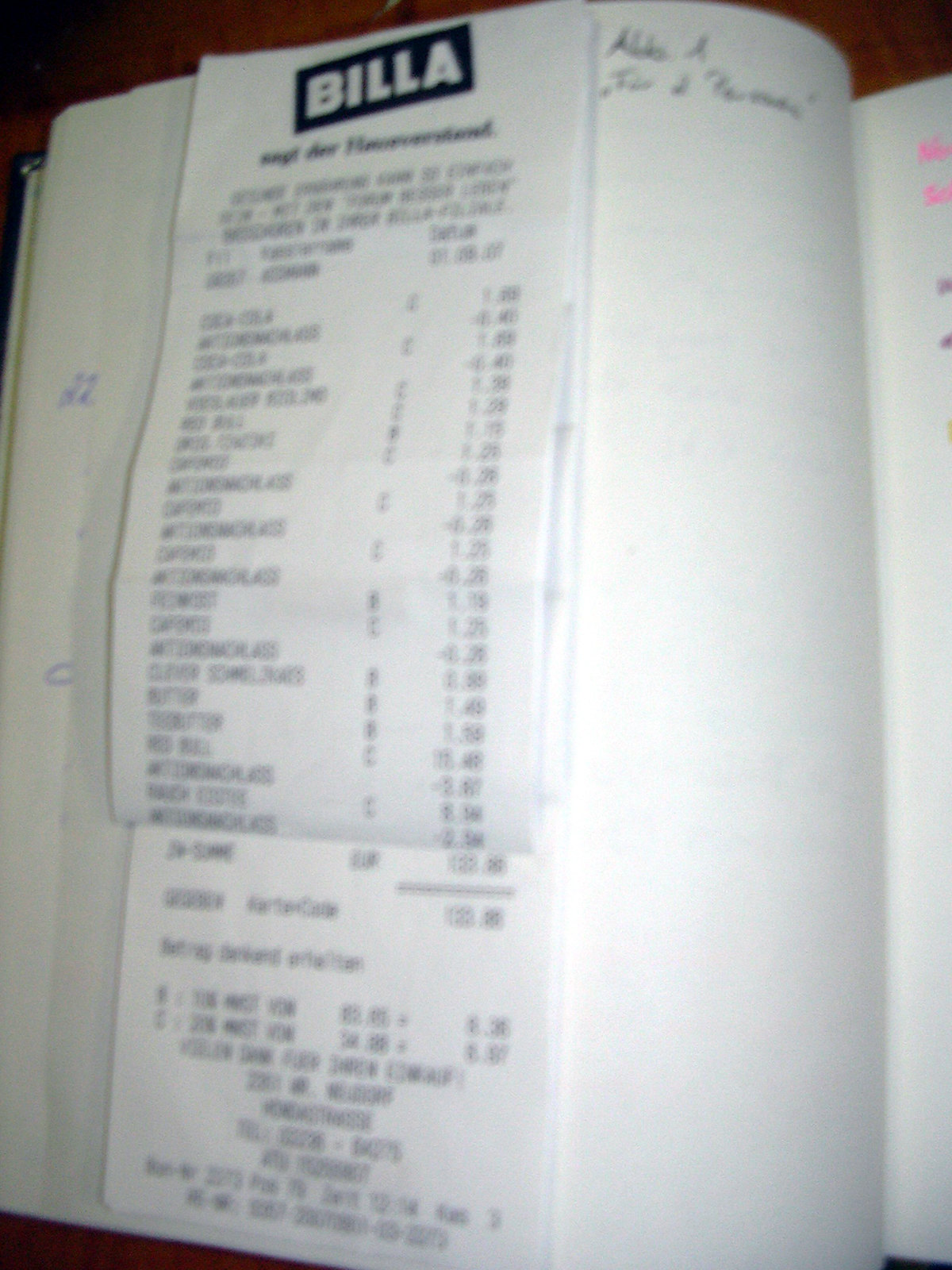An unfolded, lengthy white receipt from BILLA, prominently displaying the store name in bold white letters against a black background (B-I-L-L-A), lies atop an open book with white pages. The receipt features a series of itemized entries, each listing items on the left, accompanied by corresponding numbers on the right. The open book beneath the receipt is filled with handwriting in various colored inks: pink and purple writings are visible on the right-hand pages, while black and blue writings adorn the left-hand ones. The book appears to contain some blank pages as well. This entire setup rests on a brown-colored surface, likely a table.